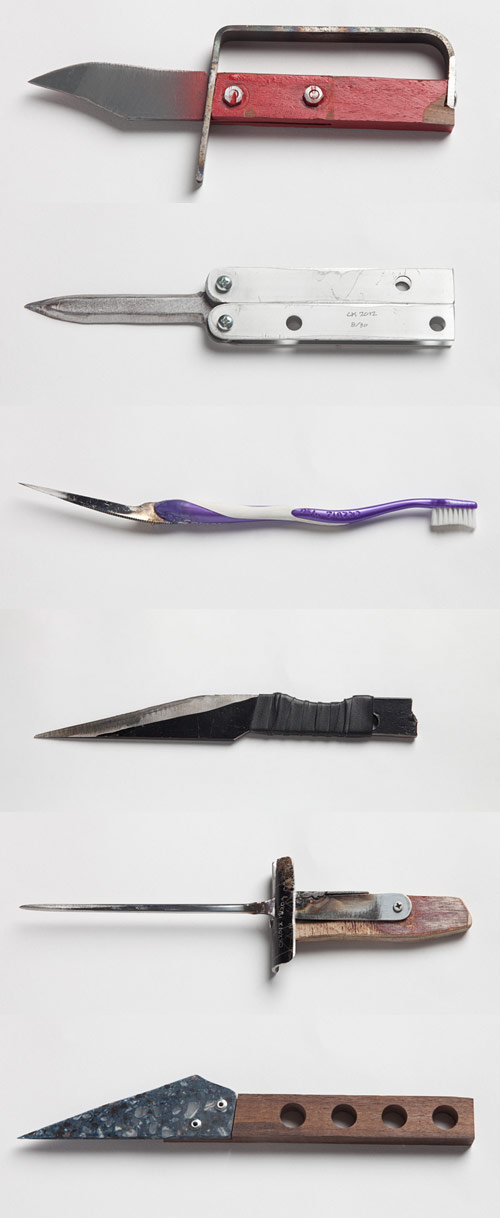This image showcases a collection of six distinct knives lined up vertically on a gray surface. At the top, there is a knife with a red handle, featuring a red hand guard and a silver blade. Below it, a silver butterfly knife stands out with its sleek design. The third knife down resembles a toothbrush, with a purple and white handle and a sharpened blade where the bristles would be. Next, there is a compact knife, entirely metallic in appearance, its handle wrapped in cloth. Following that, an ice pick-like knife with a very thin, almost needle-like blade and a wooden handle with a light-colored material is displayed. At the bottom of the lineup, a triangular knife features a brown wooden rectangle-shaped handle with four circular cutouts, while its gray blade appears to be made from some sort of stone. This diverse assortment highlights a range of homemade and fashion knives, each with unique characteristics and materials.